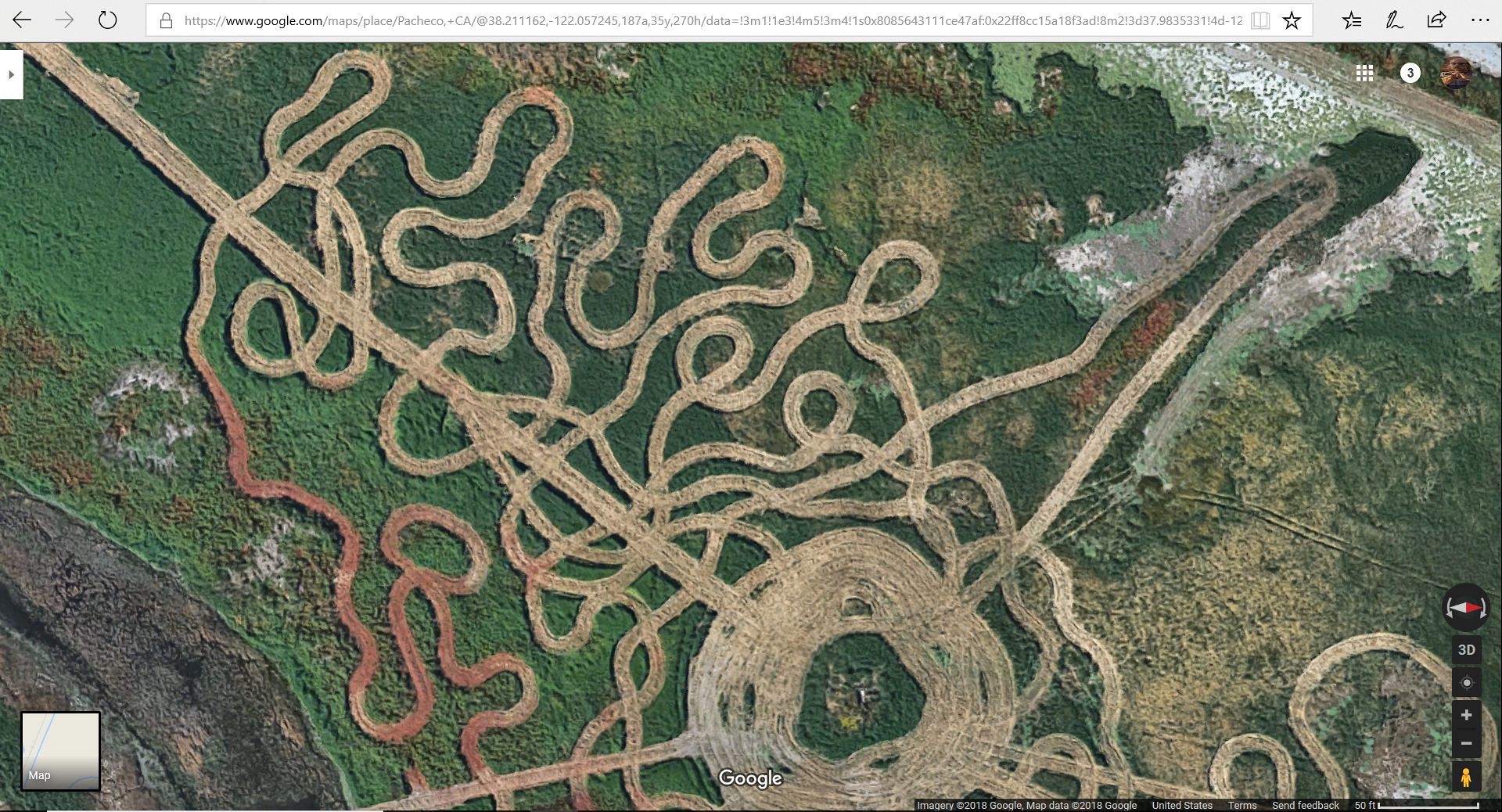An aerial shot captures what appears to be an abstract, maze-like design sprawling across a surface that resembles old concrete. The central focus is a roughly circular area filled with concentric circles and a green patch at its core. Extending outward from the center are numerous squiggly lines and flowing arcs that move in various directions, resembling yarn or wool intricately laid out. The background predominantly features green, with patches of white and khaki hues interspersed throughout. In the lower left corner, a clickable interface suggests this is part of a user interface, likely from a game map displaying surface features. Additional details include a dark rock or wall on the left, with a white cylindrical object, possibly a piece of toilet paper, adding curious texture to the scene. The entire composition is dotted with lines of varying colors from light brown to dark brown, contributing to the chaotic yet fascinating landscape.